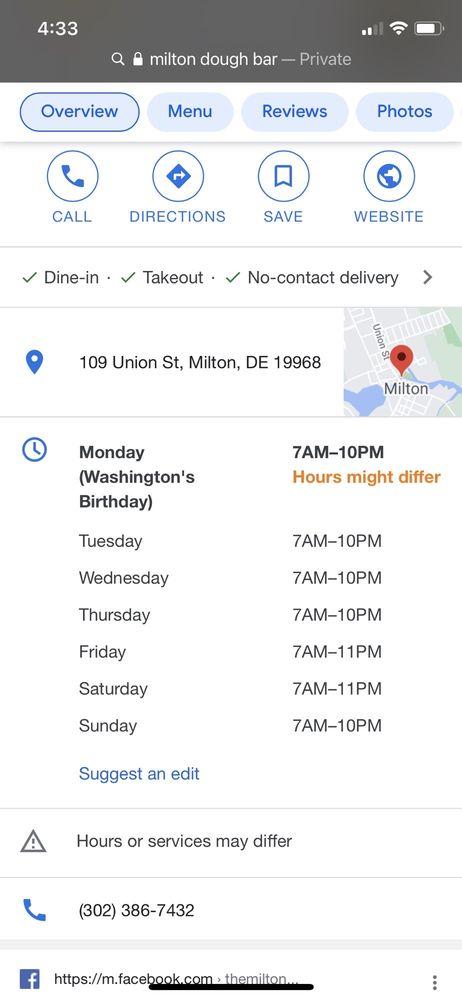This screenshot from a cell phone displays a web page for Milton Dobar. At the very top, the menu bar or URL bar is visible, featuring a dark brownish-gray color, mostly gray. The time is shown as 4:33 PM, and the battery indicator on the right shows approximately 90% charge. 

Beneath the URL bar, labeled "Milton Dobar - Private," directions to Milton Dobar are provided. Several interactive buttons are located at the top: a call button, a directions button, a save button for storing information on the phone, and a link to the Milton Dobar website. 

Below these buttons, three dining options are presented, each with a checkmark to the left: dine-in, take-out, and non-contact delivery. These options indicate the different ways to enjoy a meal at Milton Dobar.

A map occupies the next section, featuring a red pin indicating the location of Milton Dobar. To the left of the map, the address is displayed as 109 Union Street, Milton, Delaware, DE-19968.

Further down, the operating hours of the bar are listed. At the very bottom of the page, the phone number for Milton Dobar is provided, followed by a link to their Facebook page, accompanied by the Facebook logo.